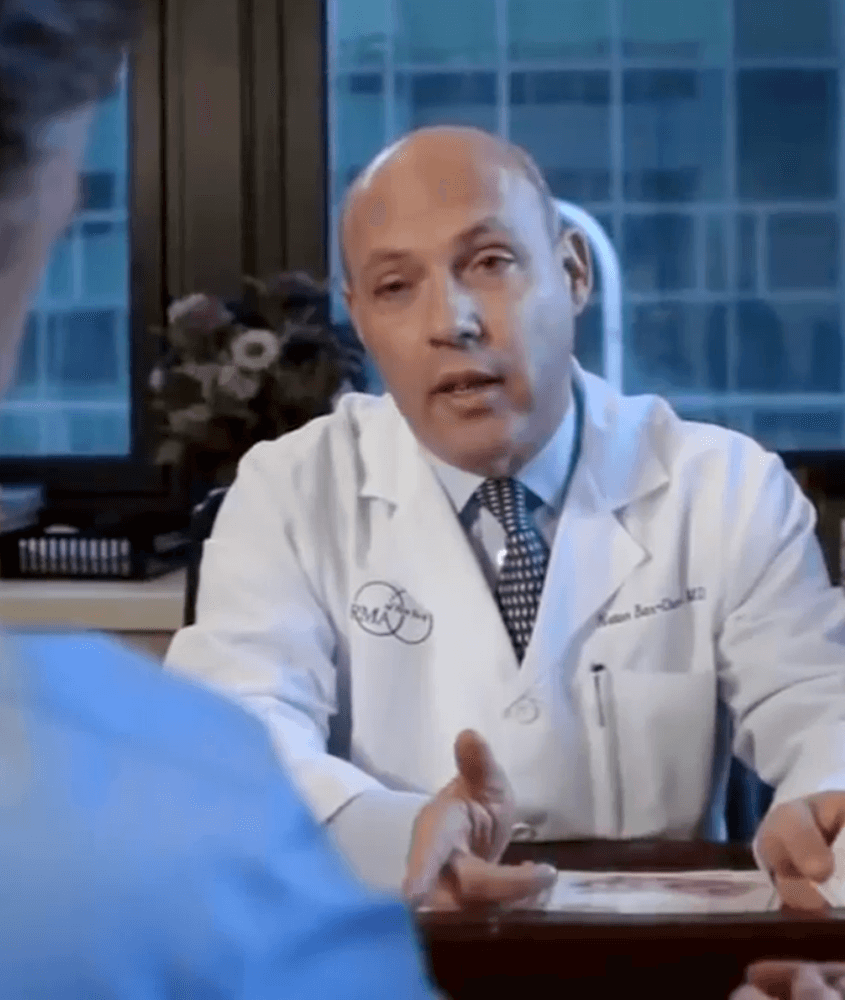The image depicts a Caucasian doctor engaged in conversation with a patient in his office. The doctor, identifiable by the "MD" on his white medical jacket, also has two interlocking circles with "RMA" on the left breast pocket. He is wearing a white collared button-up shirt with a navy blue tie featuring white dots. The doctor has a bald head with hair only on the sides and is seen gesturing with his right hand while holding a piece of paper on the wooden desk with his left hand. The setting includes a window behind him, revealing a building with bluish walls, and a flower pot on the desk. The patient, seemingly a middle-aged man with gray hair, is partially visible from behind, wearing a light blue collared shirt. In addition, another person's fingers are slightly visible near the patient, hinting at a second person present in the consultation.